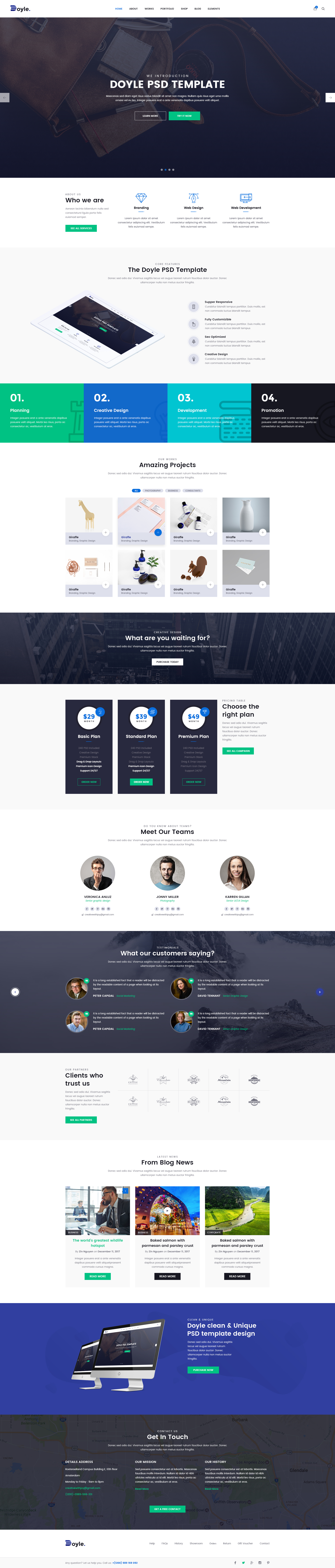This image depicts a detailed mockup of a website builder template, presumably labeled as the "Doyle PSD Template." Dominating the top of the page is a large, dark-colored rectangular banner featuring an office desktop background with indistinct objects scattered across it. Centered within this banner is bold text stating "Doyle PSD Template." Below this title, there are two contrasting buttons: a clear button with white text and a green button with white text, though the text on both buttons is too small to discern.

The template's design flows into several vertically stacked sections. At the beginning of these sections, there is a row of four colored boxes—green, blue, light blue, and black—each numbered from 01 to 04. These boxes likely serve as headers or labels for different sections of the website. Progressing down the page, multiple additional sections are prefilled with placeholder text, which would need to be customized by users tailoring the template for their own website. The detailed structure and placeholders imply functionality for various content types and suggest an intuitive layout design for a customizable website.